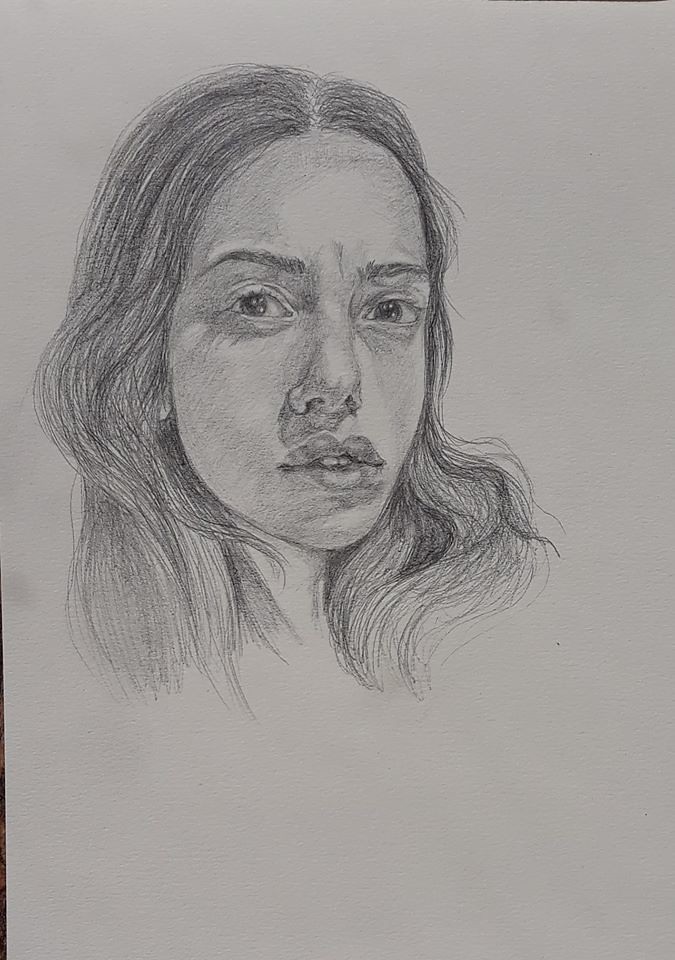This detailed hand-drawn portrait of a young woman is rendered in black and white, using either graphite pencil or charcoal on an off-white paper with a bluish-gray tint. The woman’s face is oval-shaped with long, slightly wavy, dark hair parted in the middle, cascading down to her shoulders and partially obscuring her thin, elongated neck. Her gaze is direct and intense, almost soul-searching, drawing the viewer in with a sense of deep emotion and distress.

Her facial features are meticulously detailed: full, pouty lips with a glimpse of her front teeth, prominent arched nose with elongated nostrils, thick eyebrows, and tired almond-shaped eyes. The shading is delicate but precise, giving depth to her high cheekbones and the subtle wispiness of her hair. A faint outline of her right ear is visible, adding to the realism of the portrait. The background of the paper is mostly bare, focusing full attention on the evocative expression and fine details of the woman's face.